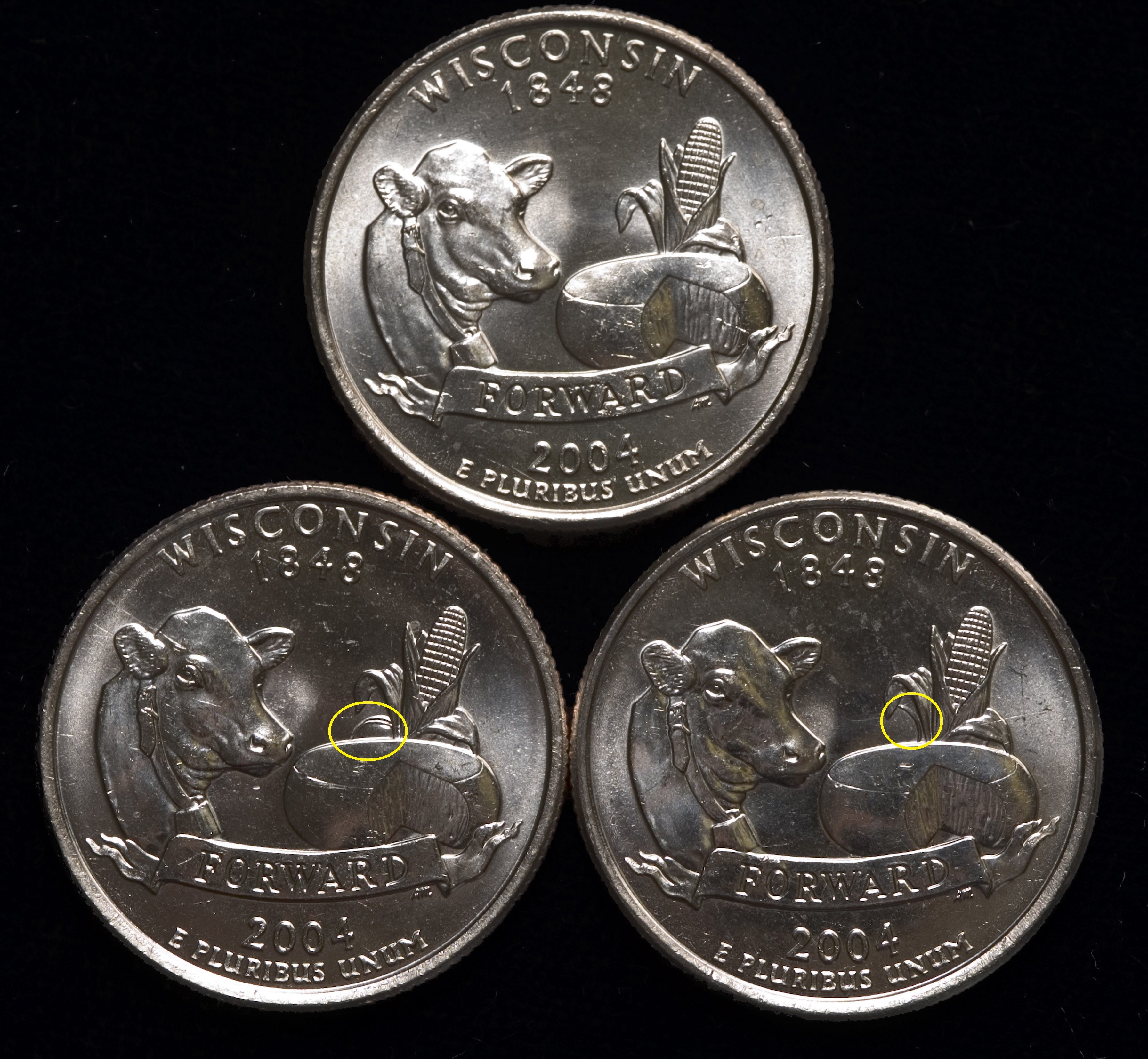The image is a color, square-format photograph showcasing three coins against a solid black background. At the very top, there's a single quarter depicting the front side, which features the word "Wisconsin" along the top border, the date "1848," a cow's profile on the left, a round of cheese to the right, and an ear of corn behind. A banner reading "FORWARD" runs across the bottom, followed by the date "2004" and the phrase "E Pluribus Unum." Below this coin are two additional quarters placed side by side, concentrating on the back. These depict the same elements but highlight a discrepancy at the bottom of the corn stalk. The left quarter has the original design, whereas the right quarter shows an additional leaf, indicating a minting error. The differences are circled in yellow for clarity.